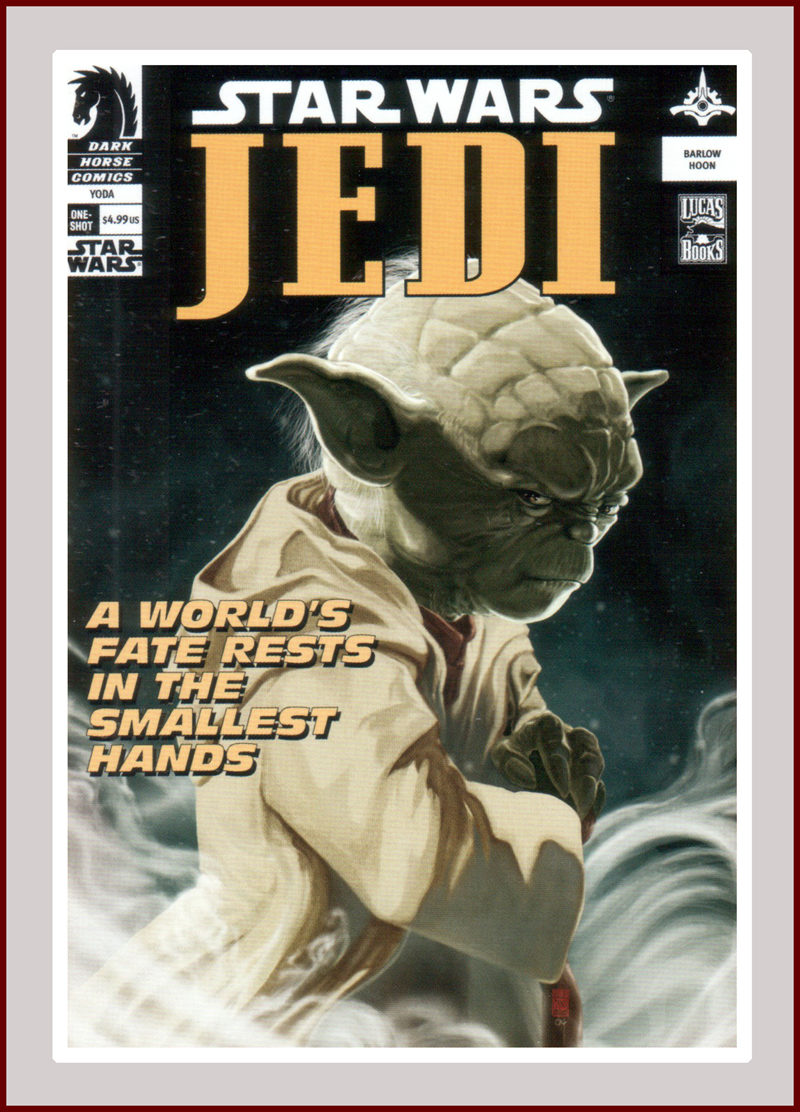This image is the cover of a Star Wars comic book titled "Star Wars Jedi," published by Dark Horse Comics. The top left corner features the publisher's logo—a black horse silhouette—alongside the price of $4.99 and the text "Yoda One-Shot." The title "Star Wars" is prominently displayed in white, with "Jedi" in bold orange text below it. The upper right corner bears the logos of Lucas Books and Shadow Moon.

The central image is a detailed, painted depiction of Yoda. He is shown in a side view, wearing his usual brown robe and holding a small, brown wooden cane. His face displays a stern expression, with shadows casting a dramatic effect. Around his feet, there is a swirling fog or smoky mist. The background of the cover is dark, adding to the mysterious and intense atmosphere. A caption near the center of the image reads, "A world's fate rests in the smallest hands," emphasizing Yoda's significant role. The overall artistic style of the cover is painted, giving it a classic and striking appearance.